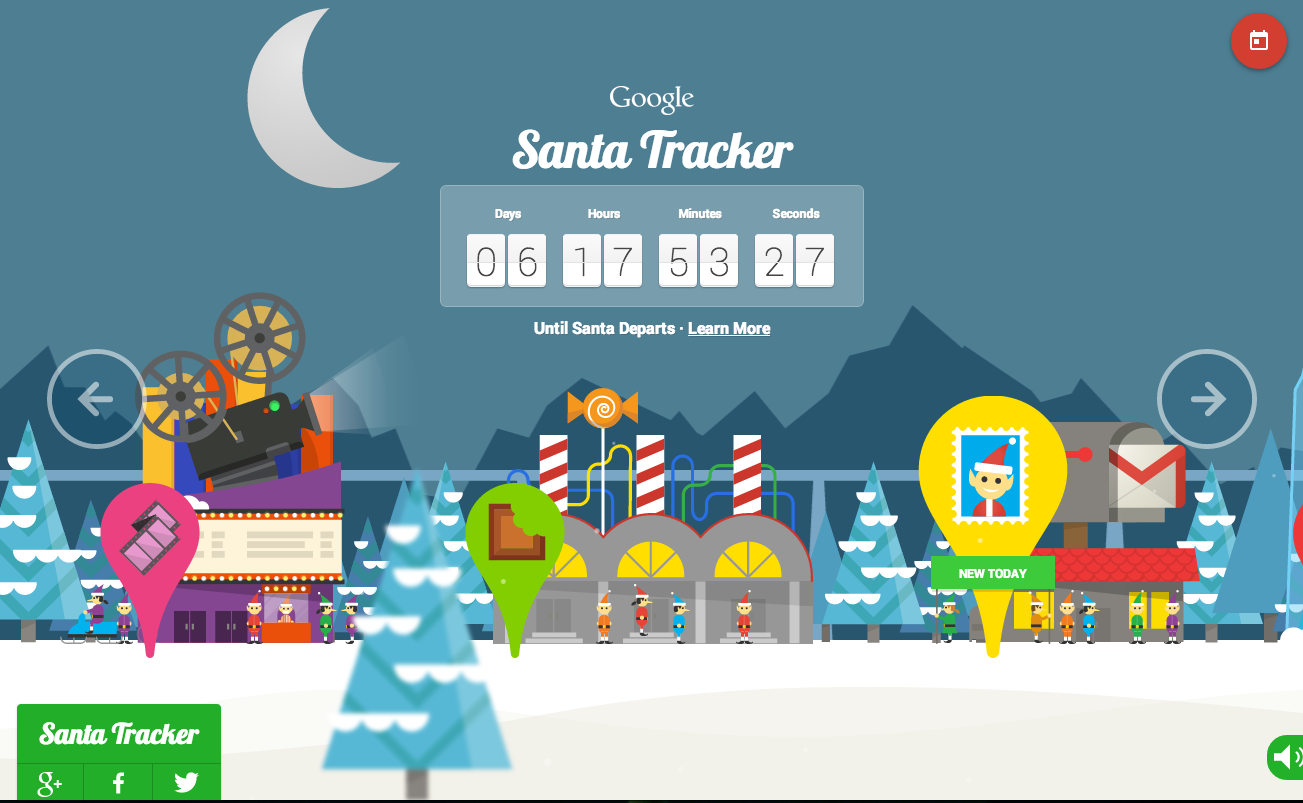This is a detailed screenshot of the Google Santa Tracker interface. The screen prominently features the Google logo in white text, followed by "Santa Tracker" written in a cursive white font. A crescent moon can be seen in the top left corner against a medium blue sky, which serves as the animated background.

In the distant background, animated mountains are visible, while the foreground showcases a festive village scene. Various buildings and elves in colorful suits—purple, blue, orange, and green—populate the scene. On the top left, a building resembling a movie theater stands out with an old-fashioned movie reel and camera icon above it. 

Scattered around the village are animated trees adorned with snow, depicted in blue and white. In the middle of the scene, there's a building that appears to be a factory, marked by a green Google Maps pin. A purple pin marks the movie theater, and a yellow pin with an elf smiling and a postage stamp indicates a new feature, accompanied by the text "I'm new today."

Next to this building, a large mailbox with a piece of mail sticking out enhances the festive ambiance. At the center-bottom of the image, directly beneath the "Santa Tracker" text, there's a rectangular countdown box displaying the time remaining until Santa's departure: 06 days, 17 hours, 53 minutes, and 27 seconds. Below the countdown, the text reads "until Santa departs," with a clickable "Learn more" link.

In the upper right corner, a red circle icon featuring a calendar is visible, while the bottom left includes "Santa Tracker" with icons for Google+, Facebook, and Twitter. The bottom right corner has an icon for toggling volume on or off.